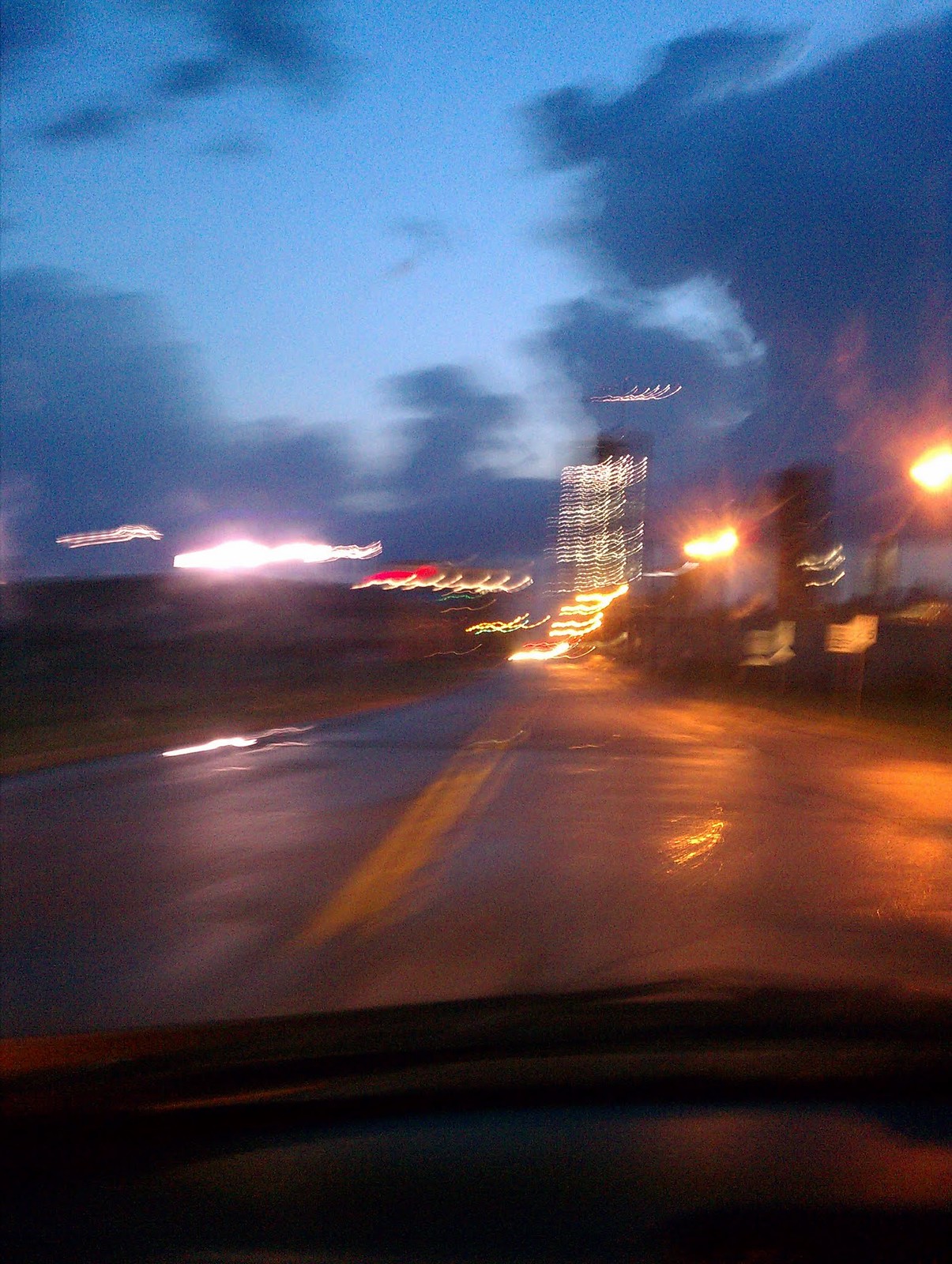This photograph captures a rainy evening scene from the inside of a vehicle. The interior features a dark gray to black dashboard, partially visible. Through the windshield, the wet street stretches ahead, marked by water slicks and illuminated by ambient streetlights. A prominent yellow line runs along the pavement, which reflects the diffuse lights, adding a glistening effect. In the background, a skyscraper stands tall, subtly highlighted by a soft amber glow from nearby lights. Street lamps dot the scene, casting a gentle warm light. The sky, painted in shades of bluish-gray, harbors dark clouds, enhancing the moody atmosphere. Patches of green grass are visible on the roadside, accompanied by several street signs bearing white and black designs. Distant car headlights pierce the twilight, contributing to the urban landscape. Though the image is slightly grainy and somewhat out of focus, it still maintains commendable quality, capturing the essence of a serene yet bustling cityscape on a rainy night.